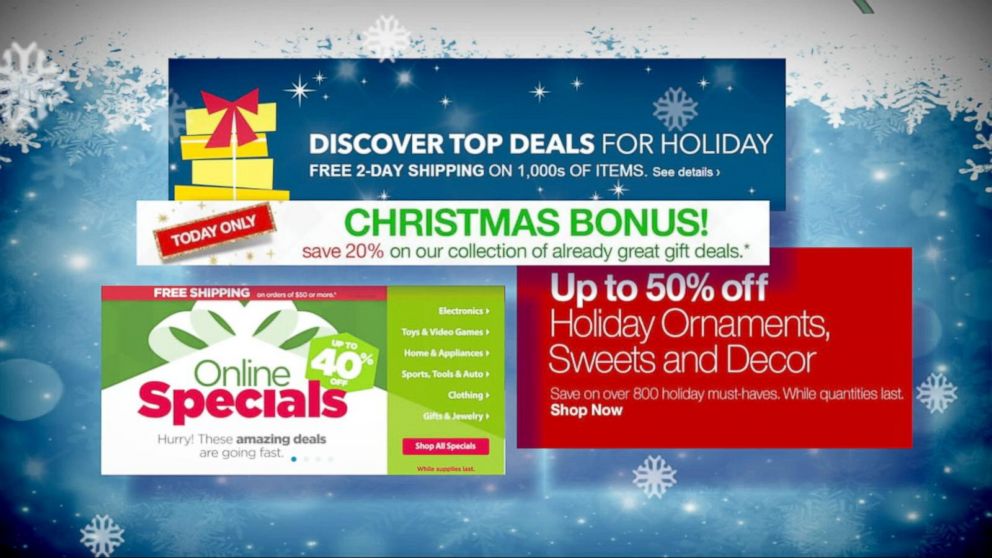The image is a screenshot of what appears to be an advertisement, although it is unclear whether it is displayed on a computer screen or a TV. The background features a winter-themed landscape with varying shades of blue and gray, adorned with numerous snowflakes scattered throughout.

In the foreground, there are three long rectangular advertisement boxes arranged in a vertical column. The first box at the top has a blue theme and contains text promoting holiday deals, specifically mentioning "Discover top deals for holidays," "Christmas bonus," and "Free two-day shipping." 

The second advertisement box is positioned below the first and stands out with its green and pink hues. It advertises online specials, highlighting "40% off with free shipping."

To the right and slightly overlapped by the top box, the third advertisement box is entirely red and promotes discounts on holiday items. It boasts "Up to 50% off holiday ornaments, sweets, and decor."

All three advertisement boxes seem to float against the snowy background, with the top box slightly overlaying the red box. The entirety of the scene is punctuated by abundant white snowflakes and dots, enhancing the festive atmosphere.